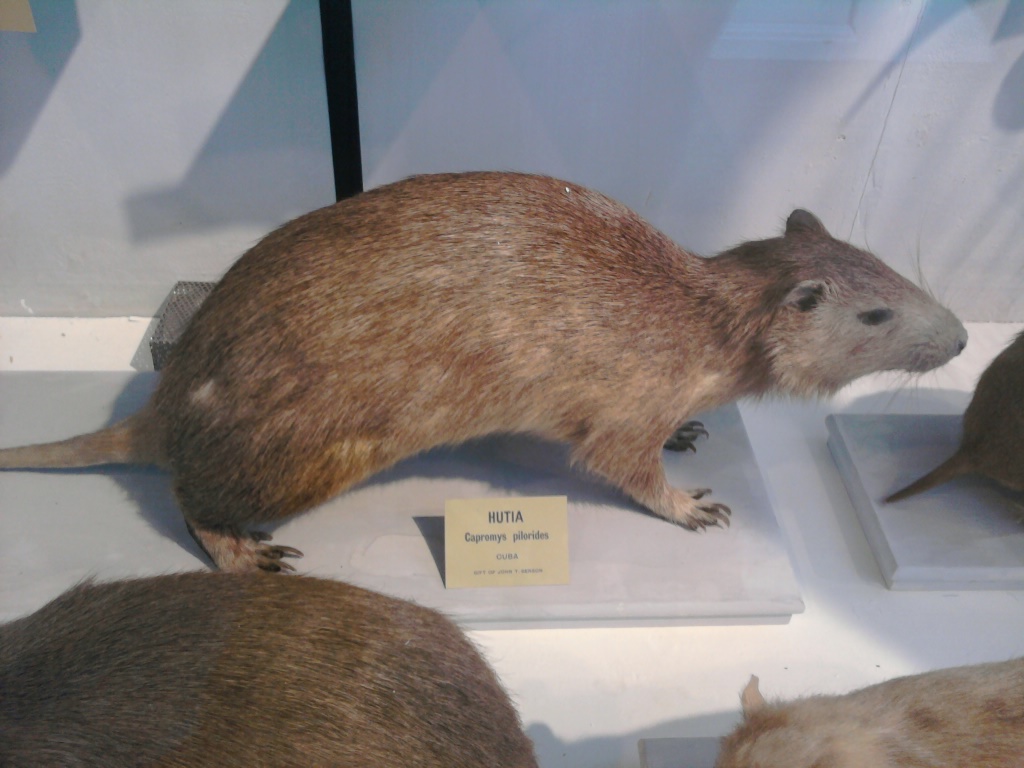The image features a taxidermied Hutia, a relatively large rodent native to Cuba, prominently displayed in a museum setting. The Hutia, which has brownish and lighter brown fur, notably resembles an oversized rat. The display includes other, partially visible stuffed rodents: one to the right and two towards the bottom. The exhibit is set against a white backdrop. Accompanying the Hutia is a yellow name tag that reads "Hutia" above its Latin name, possibly "Capronis Pillarides," and below them, the word "Cuba."